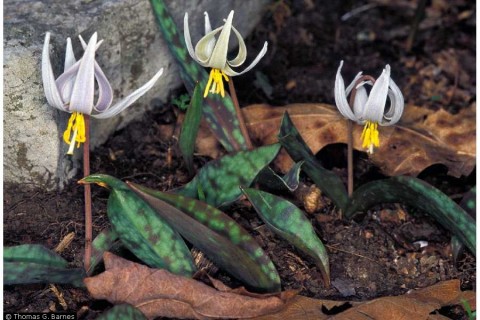The vivid photograph captures a close-up of three unique flowers emerging from the soil, each possessing thin, light-colored petals with striking yellow stamens and pistils that droop downward. The flowers, sharing similarities, vary slightly in hue; the left one hints at a purple shade, the middle has a tinge of green, and the right one appears gray. They all rise from brown stems amidst a scene of rich, multi-textured earth.

Around the flowers, the ground is covered with a mix of green leaves, interspersed with some brown, trampled foliage, and a few vibrant green leaves exhibiting black veins and brown mottling. The dirt appears somewhat muddy, suggesting potential moisture in the area. Adding to the natural tapestry, a large, moss-covered rock occupies the upper left-hand corner, while other smaller rocks are scattered about. The backdrop features some concrete, contrasting with the natural elements, hinting at a garden setting or a shaded forest floor.

The detailed colors and textures of the leaves and flowers create a mesmerizing display, with the scene completed by a subtle signature in the lower left corner, reading "© Thomas G. Barnes."